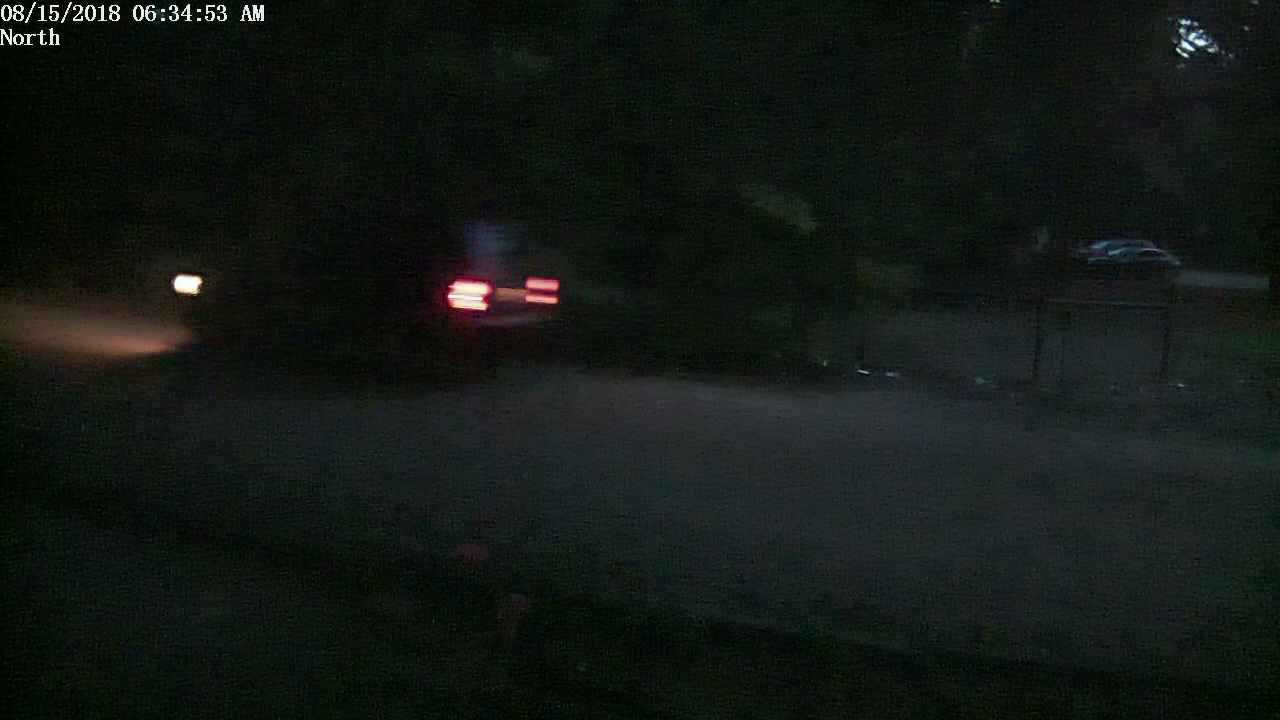This color snapshot, captured by what might be a traffic camera, is extremely blurry and taken at night. The image is dominated by a road scene. In the upper-left corner, there's a timestamp in white lettering reading "8-15-2018, 6:34:53 AM," along with the direction "North." At the center left of the photograph, there is a blurry vehicle, distinguishable by its bright white headlights casting a splash of light on the road ahead and red taillights at the rear. To the right of the vehicle, in the distance, several parked cars can be vaguely seen, possibly in a driveway or a parking area. Further ahead on the road, a poorly defined fence and yard are visible next to the roadside, enhancing the sense of depth but maintaining the overall very low-quality resolution, which makes finer details difficult to discern.